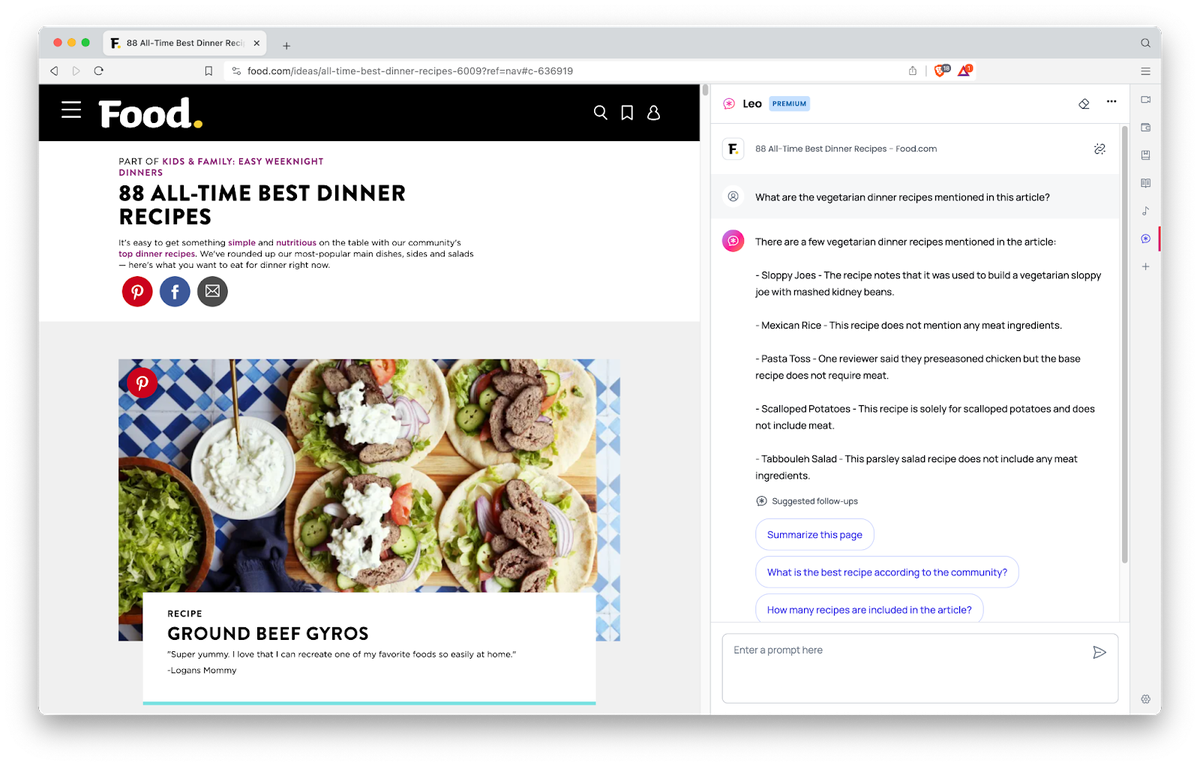This webpage from food.com prominently features the food.com logo in the upper left corner, designed with the word "food" in white letters accompanied by a distinctive yellow dot behind it. In the URL bar, the address is displayed as "food.com/deals/all-time-best-dinner-recipes-6009," with some reference rules applied.

Beneath the black banner, which also features the food.com logo, lies the main body of the webpage. The header introduces the article under the "Kids and Family" section, specifically titled "Easy Weekend Dinners: 88 All-Time Best Dinner Recipes." Directly below this header, users find social media buttons allowing them to share the article on Pinterest, Facebook, or via email.

The first recipe showcased on the page is "Ground Beef Gyros," visually represented by an appetizing image. The photo captures four different gyro preparations, each arranged artfully on a table with the meat and various ingredients layered on soft flatbread-like buns.

To the right of the main content, the webpage lists additional meal suggestions such as Sloppy Joes, Mexican Rice, Pasta Toss, Scalloped Potatoes, and Tabbouleh Salad, offering a variety of options for easy and enticing weekend dinners.